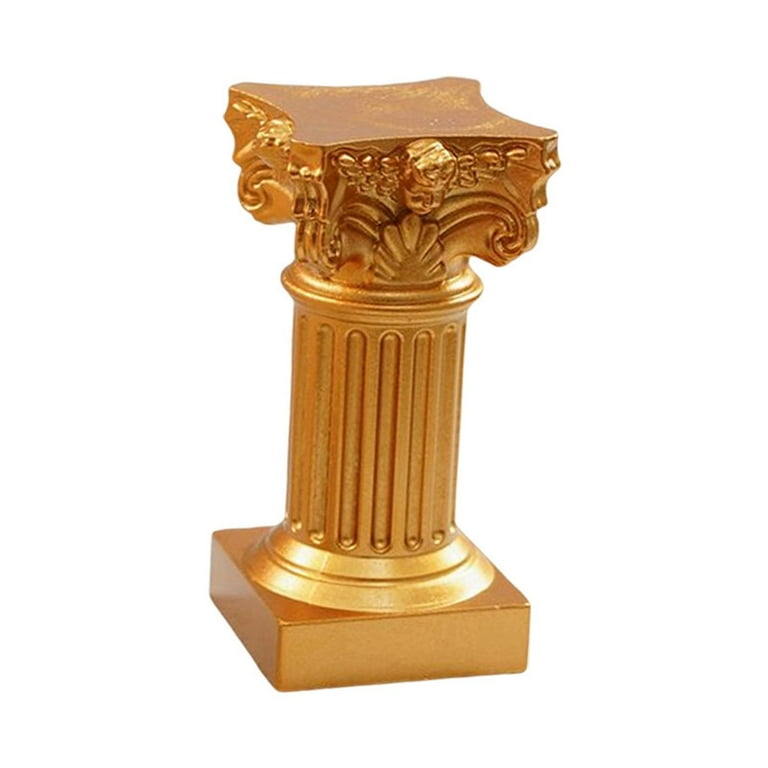This intricately staged, full-color photograph presents a vertically rectangular column that exudes a metallic sheen suggestive of a brass or gold-painted finish. The background is entirely white, making the object the sole focal point. The column stands on a slightly elevated, thick square base in a rich brown hue. Above this base, the column features a substantial, vertically grooved body that is encircled by ornate decorative elements, reminiscent of classical Greek or Roman design. These embellishments include detailed carvings resembling leaves and swirls, and prominently display cherub figures. At the top, the column narrows into another brown, flat square platform, suggesting it may function as a pedestal. This platform, coupled with the column's decorative richness, indicates the piece’s artistic complexity and potential utility in holding small objects.